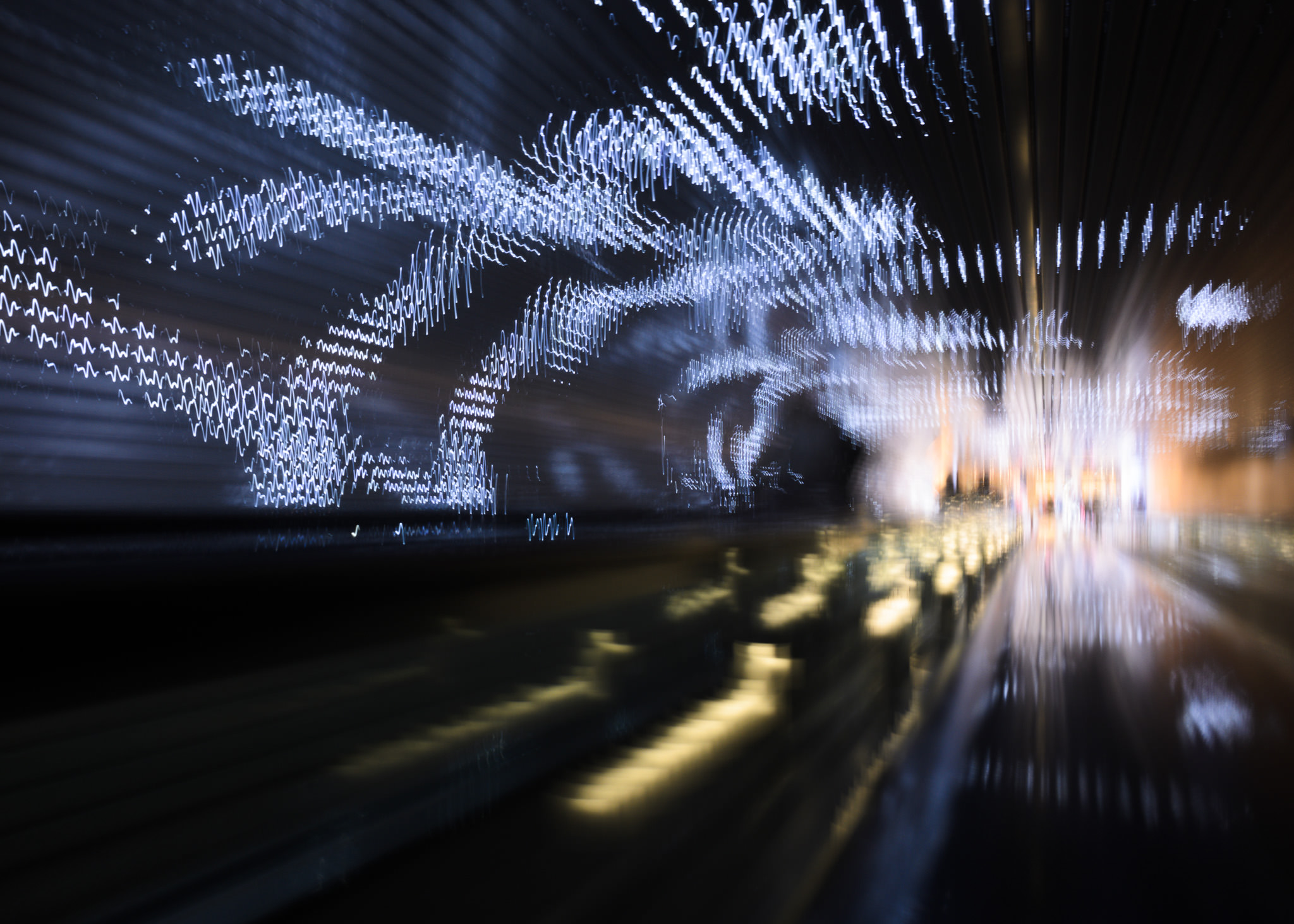The image depicts an environment reminiscent of an airport, featuring side-by-side escalators or conveyor belts moving in opposite directions. The scene is viewed from one end of the conveyor belts, tilted slightly towards the left wall. The photo is steeped in an artistic blur, likely caused by a low shutter speed and camera movement, rendering most details indistinct. However, where light penetrates the tunnel, it illuminates portions of the conveyor belts' guardrails and the floor. 

The tunnel's walls, composed of a semi-transparent glass, display a peculiar pattern of lights that form what appears to be squiggly, palm tree-like shapes. These abstract light figures run along the walls, contributing to the notion of an otherworldly or vaguely Matrix-like atmosphere. The photo's light sources, including a bright, almost sun-like glow at the far end of the tunnel, contrast sharply with the dark, nighttime-like upper portion of the image. This stark lighting creates a captivating effect, with streaks of white and orangey-peach light cutting through the scene, enhancing the surreal and mysterious quality of the photograph.